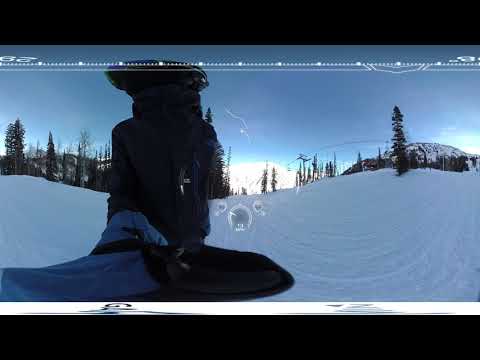The image depicts a winter scene likely at a ski resort, showing an inclined snow-covered slope with a few dark scratches and dots, and white writing that suggests it may have been captured from a computer screen or film. In the foreground, prominently, is a large black backpack with a blue sleeping bag attached, lying on the snow-covered ground, resembling someone turned away but without a person. The slopes stretch upward to a darker blue sky where the sun, possibly setting, illuminates the scene with a bright white light in the center. Flanking the slope are numerous trees, predominantly pines, and to the right, a tall, snow-capped mountain stands against a gradually darkening blue sky. The structure of a ski lift can be discerned with its cables and posts, adding to the resort-like ambiance.